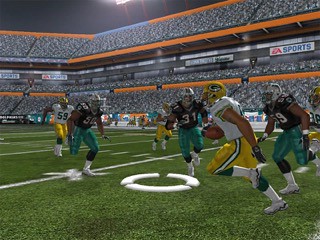The image appears to be a scene from an EA SPORTS video game. In the upper right corner, the logo "EA" is prominently displayed in red letters, followed by the word "SPORTS" in bold, blue, all caps text against a white background. 

The lower part of the image showcases a meticulously designed football field with what looks like artificial turf, though it could be a realistic imitation of real grass. Centered in the scene is a player wearing the Green Bay Packers helmet, adorned with the team's logo. The player is also dressed in the team's signature uniform, featuring yellow pants with a stylish dark green stripe running from the waist to the knee, bordered by a yellow band, or alternatively, two green bands with a yellow band in between.

Additionally, several other players are visible on the field, and in the background, you can see a large crowd of spectators in the stands, illustrating a well-represented, lively stadium atmosphere.